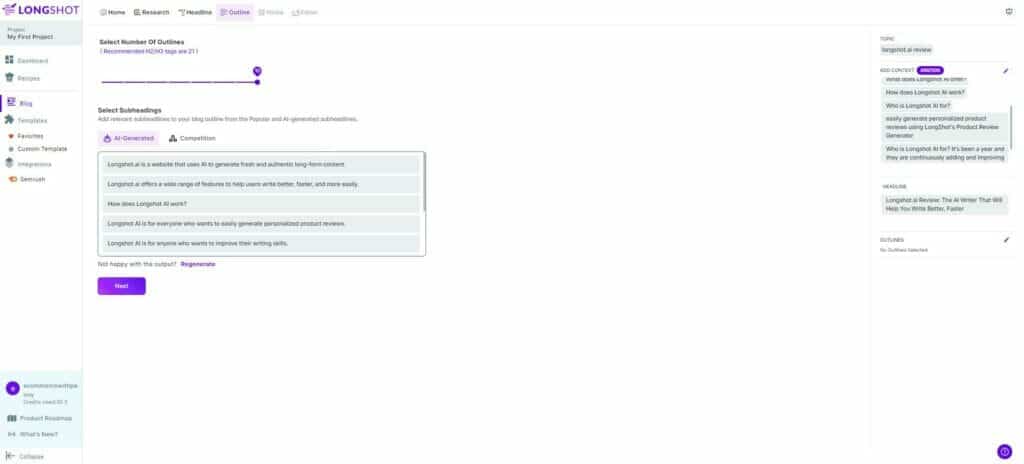This screenshot showcases the Longshot AI platform, designed for generating content and outlines. The interface prominently features the creation of a new project and the selection of subheadings for the content. On the left side, despite the blurriness, the Longshot AI logo is discernible, followed by the navigation menu with options like Dashboard, Recipes, Blog, Favorites, Custom Template, Integrations, Examples, and Community.

Central to the interface is a progress bar indicating the selection of subheadings, which allows users to add relevant headings to their content outline. The workspace is divided into two tabs: "AI Generated" and "Competitors," both purposed for subheading selection. A list of AI-generated subheadings is visible, highlighting Longshot AI's capability to generate fresh and authentic long-form content. The platform boasts features designed to help users write more efficiently and effectively. Annotations mention that Longshot AI can assist anyone in creating easy product reviews and improving writing skills. Despite the overall clarity being compromised, these key elements are identifiable within the screenshot.